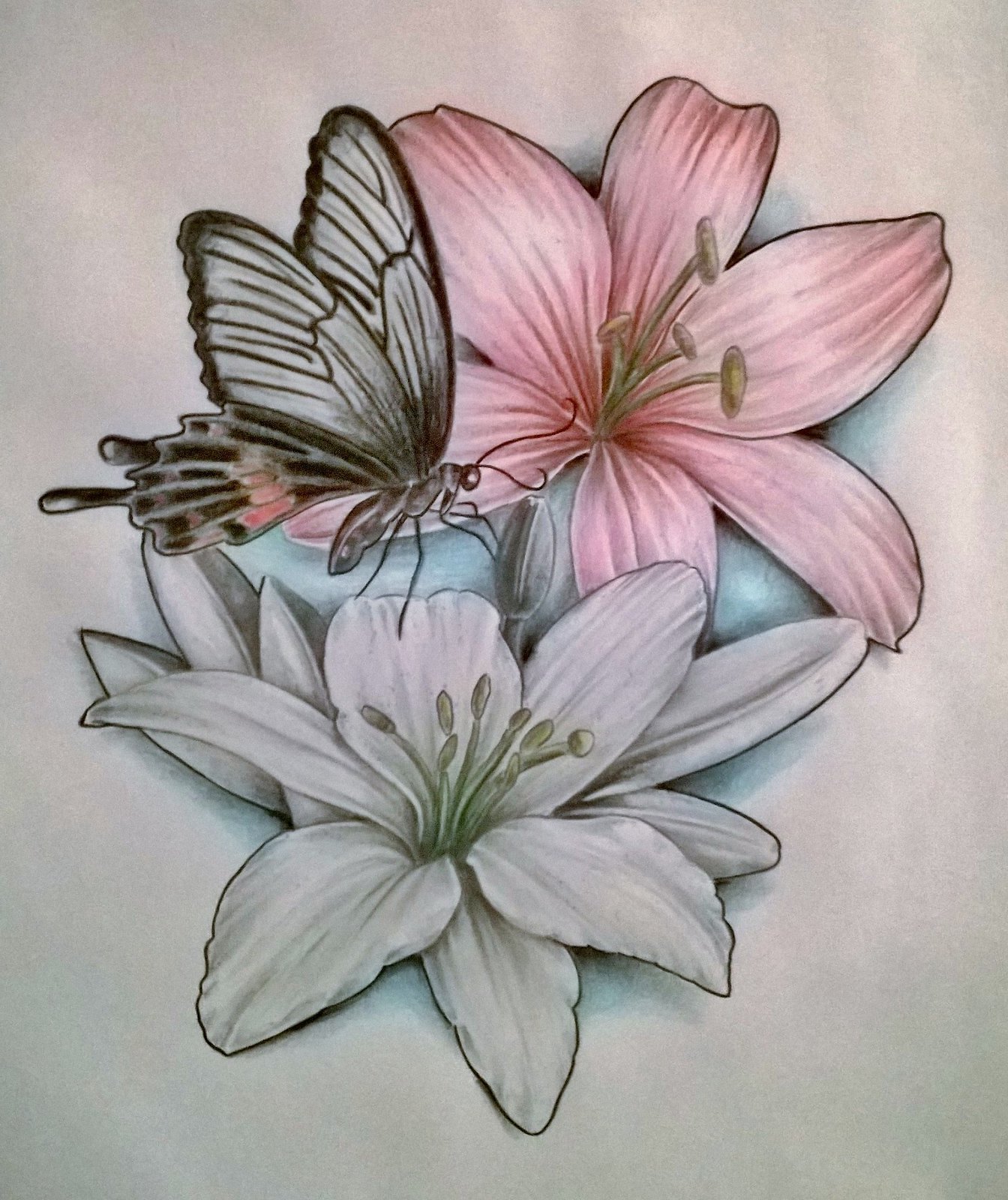This photograph showcases a detailed painting on a white canvas, featuring two prominent flowers accompanied by a black and white butterfly. The flower at the bottom has large white petals accented with blue and marked with black outlines. Its center is green, with stout green stems sprouting from it, topped with green bulbs. The upper right flower, predominantly pink with streaks of darker pink and white, also has a green center and green stems. Between the two flowers, there is a noticeable cyan splotch. Hovering above the white flower, the butterfly displays black wings with white sections for contrast, intricate black tail, and body. The butterfly's delicate features include curly antennas, patterned wings, and slender legs, enhancing the vivid depiction of nature in the artwork.